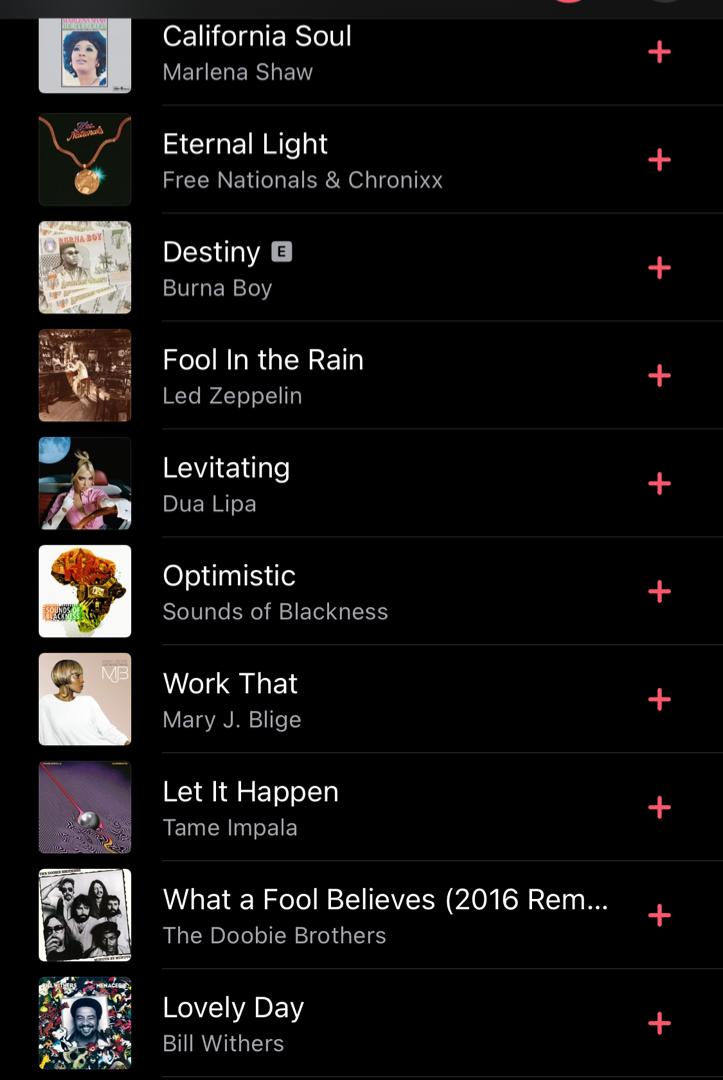The image appears to be an enlarged screenshot of a mobile app, likely Spotify, given the format and content. The background of the screen is predominantly black, featuring a list of music tracks. Each track is accompanied by a small album artwork thumbnail on the left and a red plus sign on the right, indicating the option to add the song to a playlist or library.

1. **California Soul** by Marlena Shaw - The album art is displayed on the left.
2. **Eternal Light** by the Free Nationals and Chronixx - The album logo is shown on the left.
3. **Destiny** E by Burna Boy - The letter "E" is enclosed in a rectangular button.
4. **Fool in the Rain** by Led Zeppelin
5. **Levitating** by Dua Lipa
6. **Optimistic** by Sounds of Blackness
7. **Work That** by Mary J. Blige
8. **Let It Happen** by Tame Impala
9. **What a Fool Believes (2016 remix)** by The Doobie Brothers - The remix version is indicated within parentheses.
10. **Lovely Day** by Bill Withers

Each track is neatly listed with consistent formatting, providing a clear and organized view of the music selection.